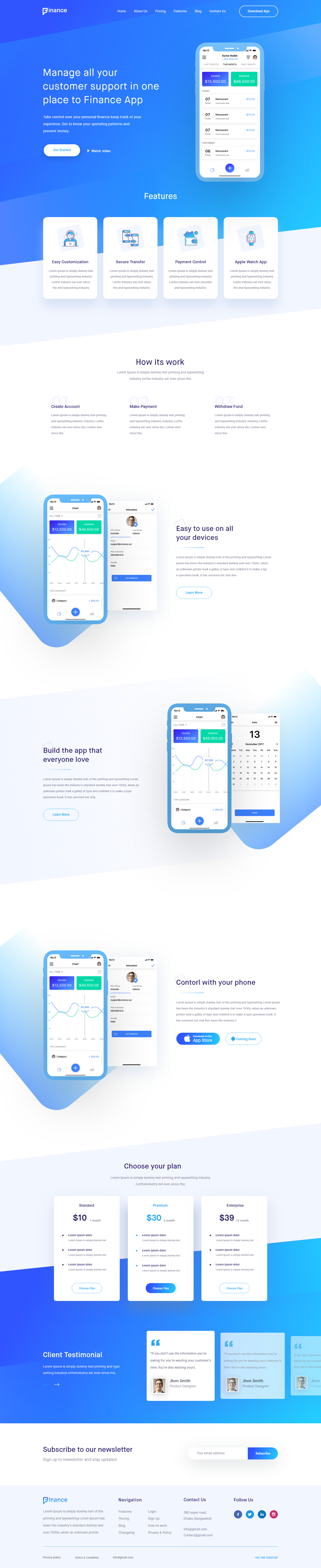The image depicts a webpage from a finance-related app, predominantly themed in blue and white. At the top of the page, the title "Finance" is prominently displayed. The navigation menu includes categories such as Home, About Us, Pricing, Features, Blog, and Contact Us. 

A notable "Download App" button is also present, emphasizing the app's tagline: "Manage all your customer support in one place with the Finance App." 

Several interactive elements are included: "Get Started" and "Watch Video" buttons, and an icon showcasing a smartphone screen. This screen displays various app sections such as "Today," "Yesterday," and a breakdown of different bills.

Under the "Features" section, the app highlights capabilities like:
- Early Customization
- Secure Transfers
- Payment Control
- Apple Watch App Compatibility

The "How It Works" section outlines three simple steps:
1. Create the Account
2. Make Payment
3. Withdraw Funds

The webpage assures that the app is easy to use on all devices and includes an image presumably representing the app’s settings interface. Another section encourages users to "Build the App that Everyone Loves," featuring a calendar and a revenue information chart.

Towards the bottom, there is a "Choose Your Plan" section with three options:
- Standard: $10/month
- Platinum: $30/month
- Enterprise: $39/month

The page also includes client testimonials and an option to subscribe to their newsletter, maintaining a cohesive blue and white aesthetic throughout.